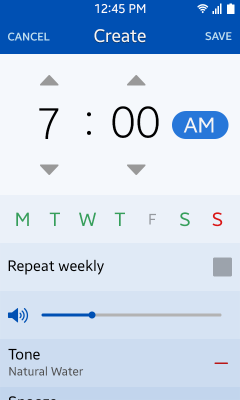This is a detailed caption for an application screenshot captured at 12:45 p.m. on a device with full Wi-Fi and carrier signal bars, as well as 100% battery life:

In the screenshot of the application, we see a user interface with a blue banner at the top, a white and light blue banner at the bottom, and various interactive elements. Dominating the blue banner in the center is a large white font text that reads "Create." On the left side of this banner, there is a "Cancel" button and on the right side, a "Save" button. The application appears to function as a clock or alarm setting utility, with "7:00 a.m." prominently displayed as the selected time.

There are gray arrows above and below the time to adjust it, supporting incremental changes. The "A.M." toggle is highlighted in a blue button. The days of the week are listed in a horizontal format, with Monday through Thursday shown in green font. Notably, Friday is highlighted in gray, suggesting it is currently being edited or selected differently. Saturday is shown in green, and Sunday is in red, indicating a different state, possibly inactive or not selected.

Below the days of the week, the phrase "Repeat weekly" is visible, confirming that the alarm is set to repeat on the chosen days. Adjacent to this is a square gray button, likely serving as an additional control.

Further down, there is a blue adjustment section for the alarm tone. It features a speaker icon with sound wave simulation emanating from it, indicating the audio component of the alarm. The selected alarm tone is described as "Natural Water," suggesting a soothing wake-up sound.